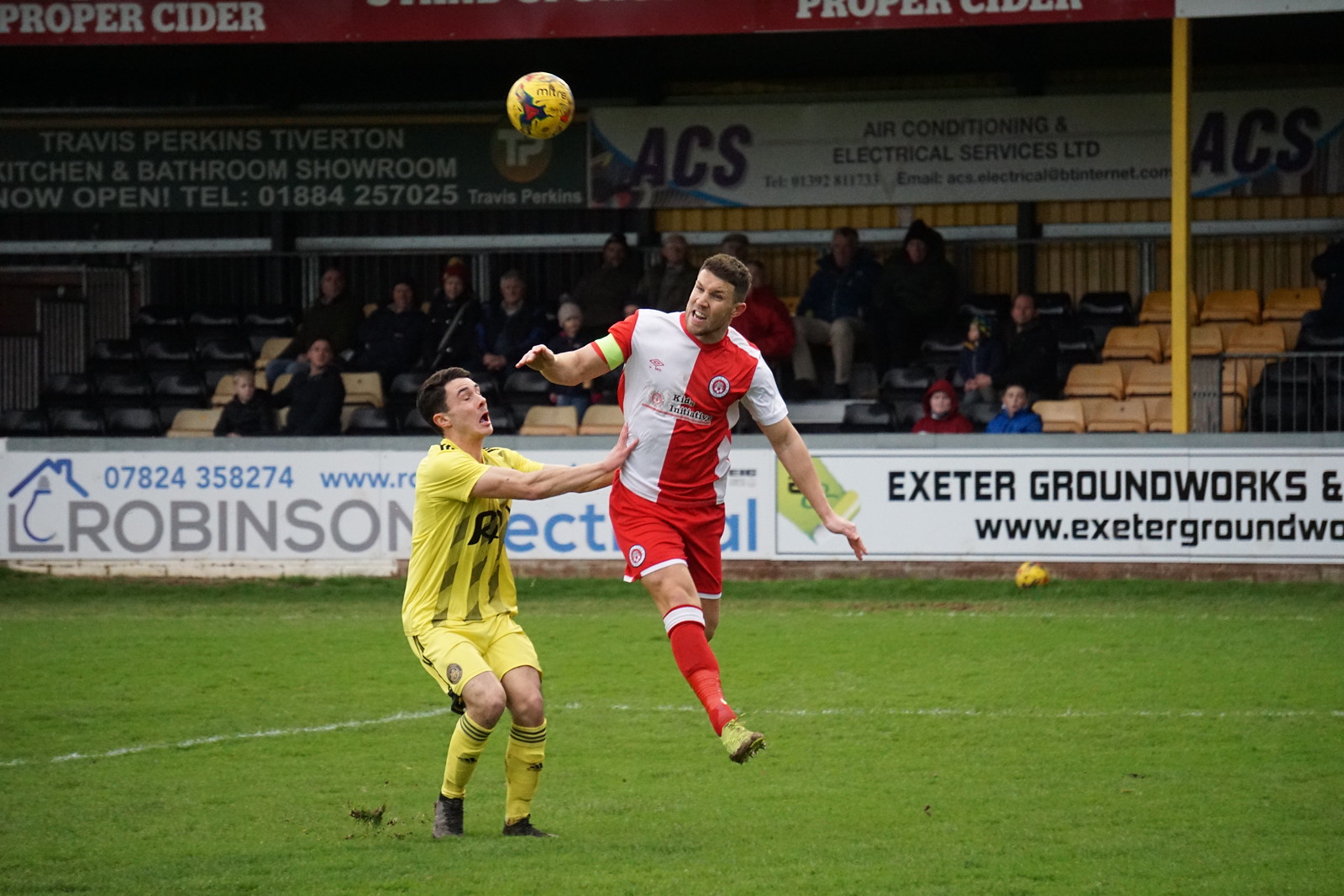In this vivid action shot taken outdoors in the middle of the day, two soccer players are captured on a large, flat, grassy field marked with painted lines. Dominating the center of the image, the athlete on the left is donned in a complete yellow uniform, comprising a jersey, shorts, and socks. His opponent to the right is airborne, evidently attempting to head a yellow soccer ball; he is clad in a striking red and white uniform, with a jersey split into red on the right and white on the left, red shorts with white trim, and red socks accented with white at the top. Notably, a yellow captain's band can be seen on his right arm. In the background, multiple rows of seating host a sparse crowd of spectators watching the game intently, interspersed with several empty seats. Flanking the stands is a wall peppered with various advertisements, including those for Exeter Groundworks and some air conditioning and electrical service companies. The scene bursts with colors such as green, white, yellow, gray, red, lime green, black, and tan, enhancing the dynamic energy of the moment.